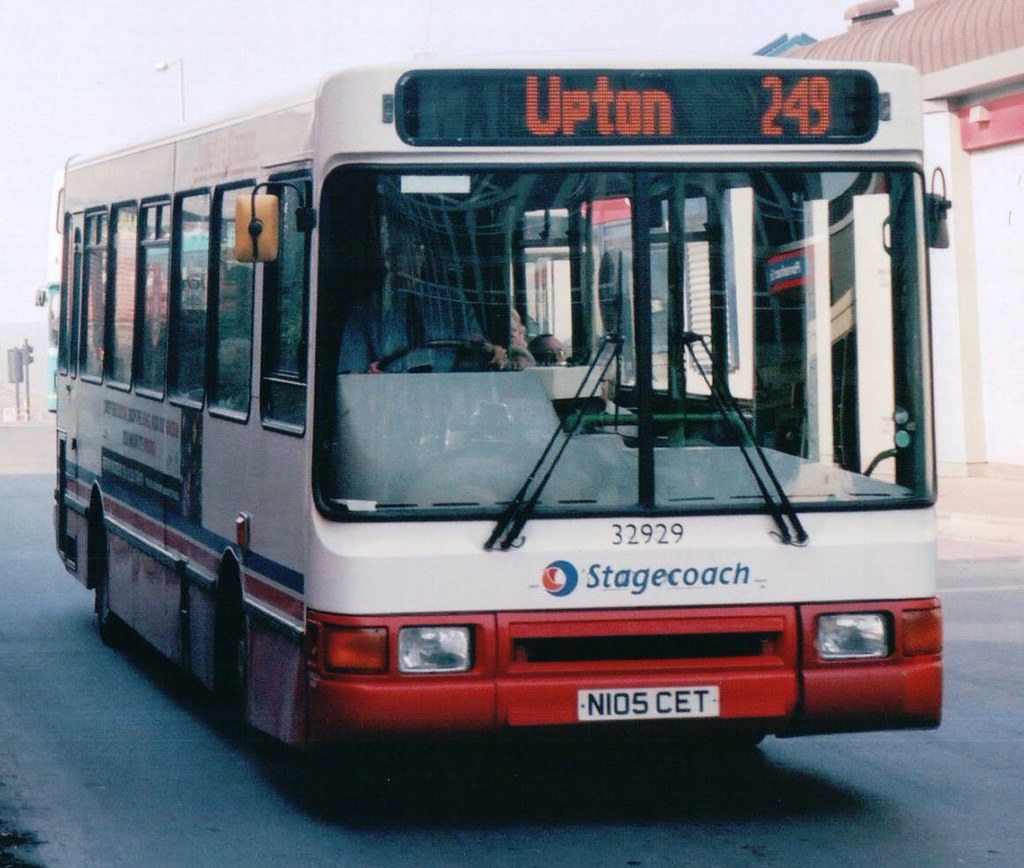The image features an older photograph of a large Stagecoach bus, predominantly white with shades of red and blue. The bus is positioned at a right-hand angle, showing both its front and right side, with seven visible windows on the right. A blue and red stripe runs along the side of the bus, above a red trim. The front bumper and area around the headlights are painted red.

Key details include a foreign license plate reading "N105CET," suggesting the bus is in Europe. Above the driver, in a large open window on the left-hand side of the bus, is a black oval digital panel displaying "Upton 249" in orange lettering. The head-on view reveals large windshield wipers in the upward position, and two large front mirrors. The number "32929" and the brand name "Stagecoach" appear prominently at the center front of the bus in blue lettering. Although slightly grainy and faded, the photograph captures a gentleman driver wearing glasses, indicating that the bus appears to be full with passengers.